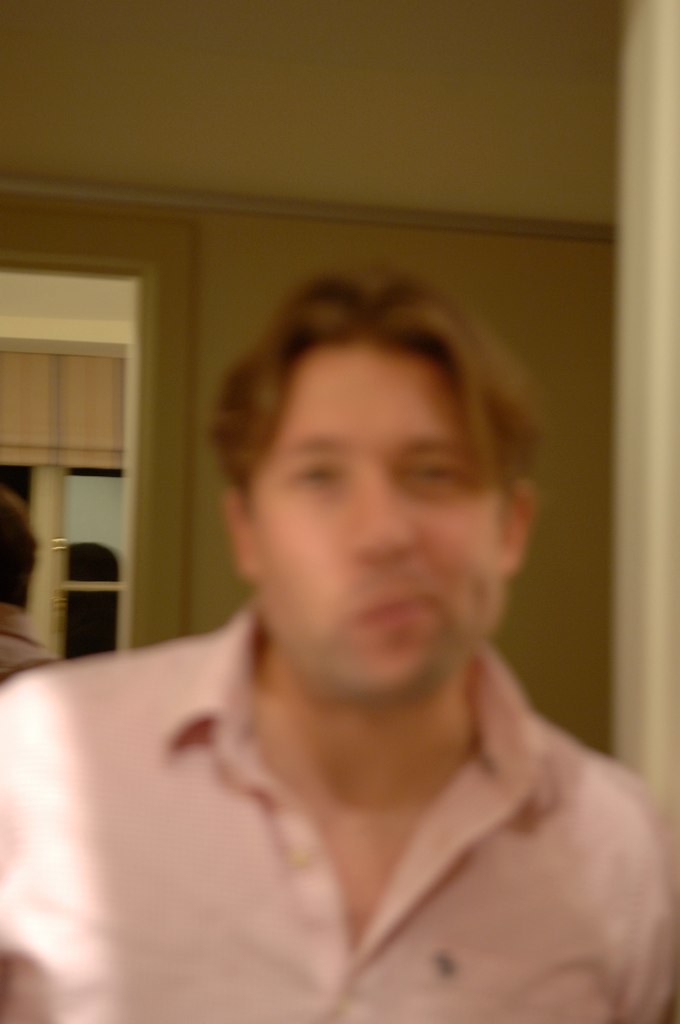This photograph features a blurry Caucasian man with short, reddish-brown hair and reddish eyebrows, standing from the chest up and facing the camera. He's making a distinctive expression, with his mouth and nose twisted to one side. The man is wearing a pink collared shirt with an unbuttoned collar and a small design on the right side. The background includes a white wall and ceiling, with an open doorway. A large mirror spans almost the entire length of the wall, reflecting the back of the man's head and his pink shirt. Additionally, there is a curtain visible ahead of him, and some areas in the background appear to be painted a dark yellowish tan.